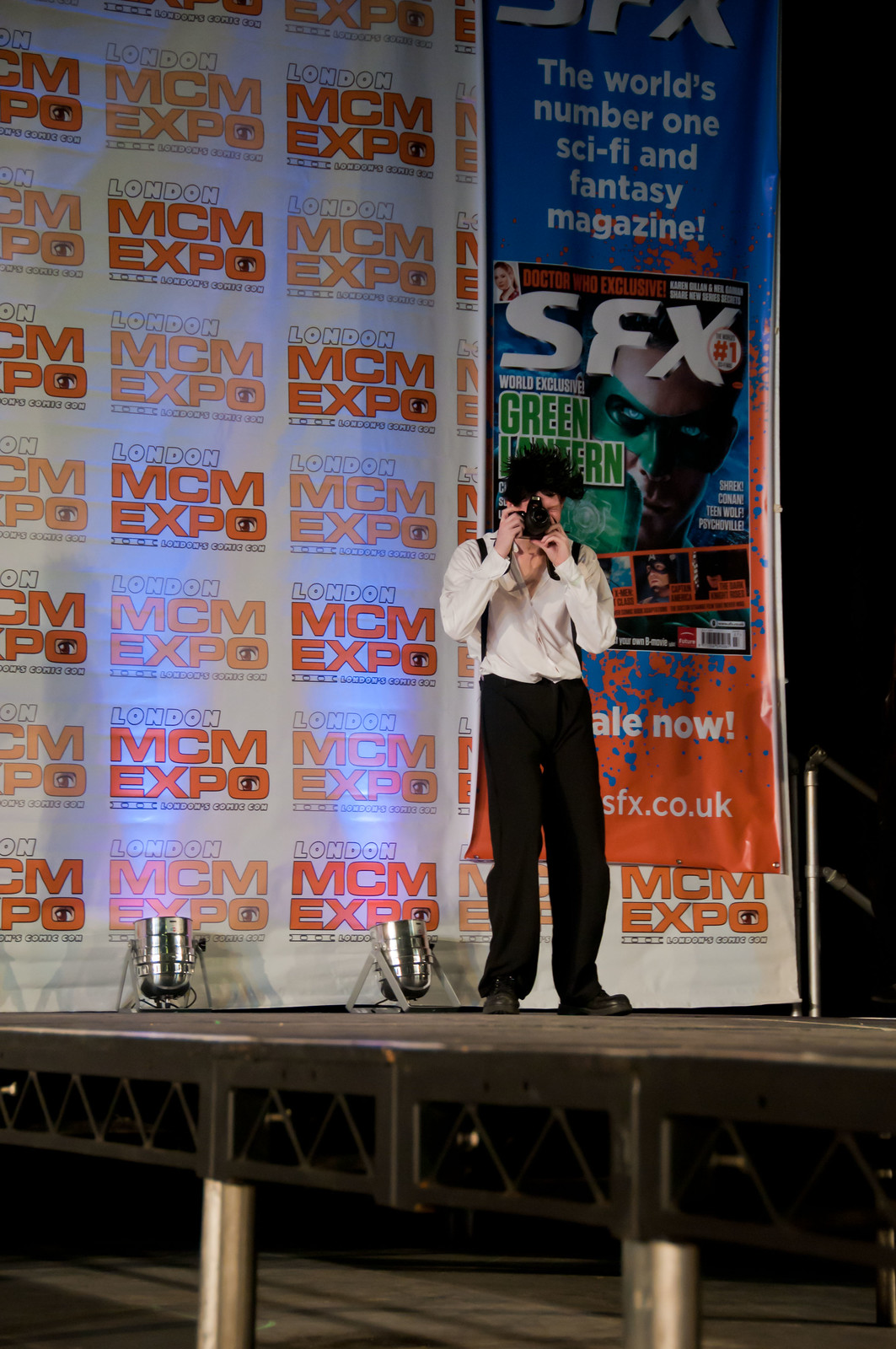The image is a detailed photograph of a man standing on a raised wooden stage with visible metal cylindrical legs, possibly above a concrete floor. The man is positioned slightly to the right of the center and is dressed in dark pants, a white long-sleeve shirt, and dark suspenders over both shoulders. He has curly black hair and holds a camera up in front of his face, preparing to take a picture.

To the left of him on the stage are two silver, cylindrical objects that could be amps or floodlights, situated on stands. Behind the man is a large white poster background plastered with repeated text, "MCM-EXPO," with a notable stylized anime eye within the "O" in "Expo". Further to the right is a banner featuring the cover of "SFX," identified as the world's number one sci-fi and fantasy magazine, adorned with various texts including references to the Green Lantern, with captions in green and orange.

The scene suggests the man is likely participating in or capturing moments at a convention or expo, characterized by the emblazoned logos and promotional materials for sci-fi and fantasy content.